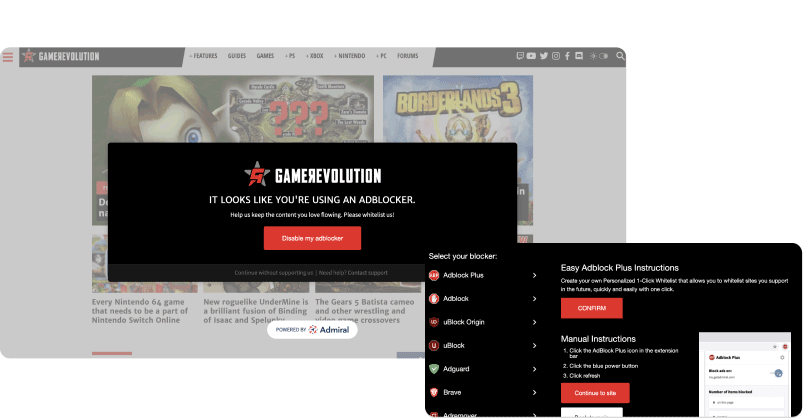Screenshot Description of Gamer Evolution Webpage with Ad Blocker Notification:

The screenshot captures the homepage of "Gamer Evolution," a website dedicated to gaming content. The page features a sleek black menu bar at the top, adorned with the Gamer Evolution logo on the upper left. The menu includes various sections such as "Features," "Guides," "Games," "PS5," "Xbox," "Nintendo," "PC," and "Forums." 

In the top right corner of the menu, there are faded-out icons for social media platforms including Twitter, YouTube, Instagram, Facebook, and Discord, indicating these options are currently inactive or de-emphasized.

A prominent pop-up notification occupies the center of the screen, warning the user about their ad blocker. The message reads, "Gamer Evolution, it looks like you're using an ad blocker. Help keep us going by whitelisting us or disabling your ad blocker." Below the message are options for "Disable my ad blocker" and a bottom right-hand section titled "Set ad blocker page," where users can select their specific ad blocker type from options like Easy Ad Blocker, Ad Block, uBlock Origin, and uBlock.

At the bottom of the pop-up, there is a button labeled "Continue to site," allowing users to proceed to the website despite the ad blocker warning. The screenshot highlights the widespread use of ad blockers among users, with some employing multiple layers of ad-blocking software.